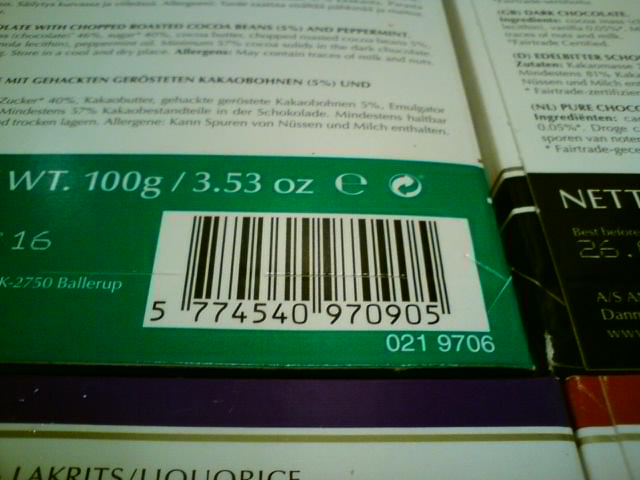This photograph captures the back of two rectangular products placed side-by-side, displaying various details prominently. The item on the left features a large green stripe with key information inscribed on it and a significant black barcode beneath it. The barcode itself exhibits the numbers "5774540 970905" followed by "021 9706". Above the barcode, the product details read "WT. 100G - 3.53oz" alongside the number "16", with "K-2750 Ballarup" positioned on the left side. This green section is complemented by a white strip with a thin gold line above it at the bottom. Multiple languages appear above the barcode area, likely listing the ingredients, but the text is mostly blurry, with only some words legible including "with chopped" and "peppermint". The product on the right showcases a black stripe instead but contains similar design elements at the bottom, with a white and thin gold strip. However, text details in this section, including several gold letterings and a mention of "licorice", remain largely illegible. The top portion of both products is a cream color.